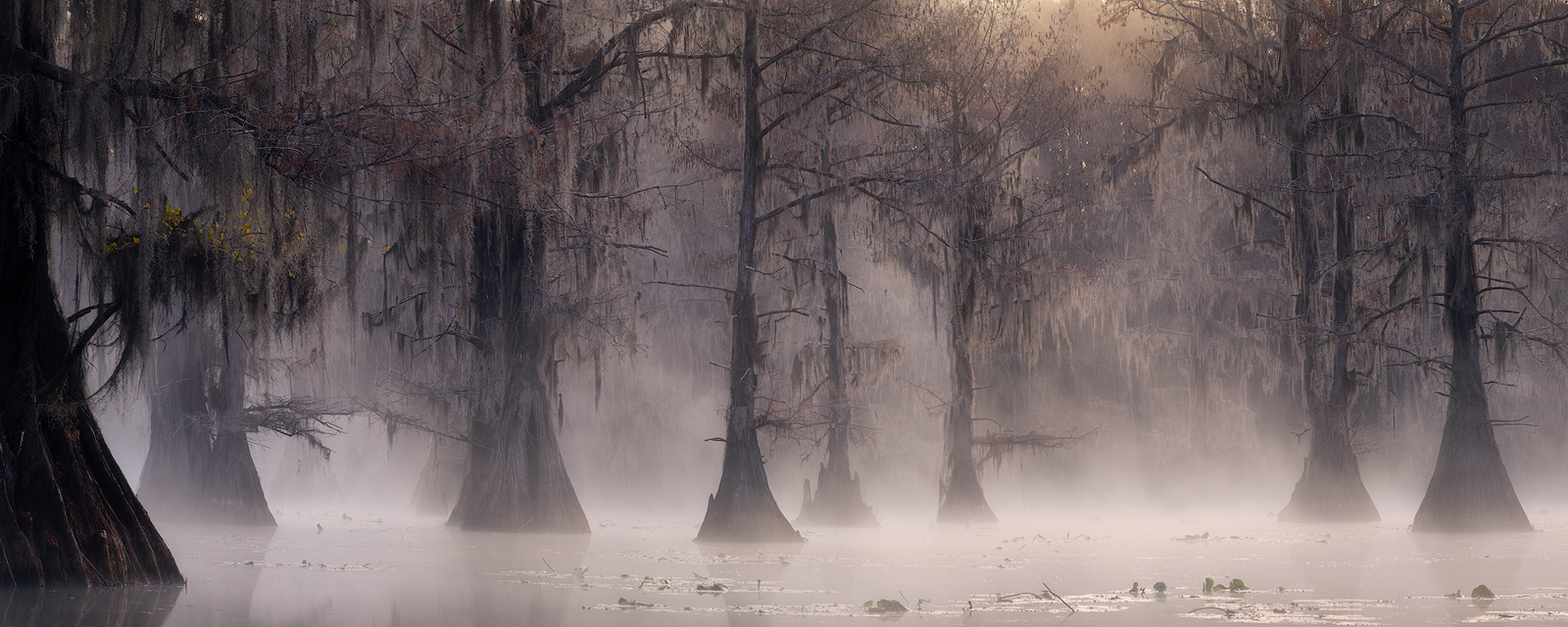This image portrays an expansive panoramic view of a mysterious, foggy swamp or mangrove forest. The rectangular image is significantly wider than it is tall, approximately three to four times in width. Dominated by a misty ambiance, the scene is filled with mangrove trees characterized by their distinctive conical root structures, which resemble teepees lifting the tree trunks above the marshy ground.

The forest floor, heavily shrouded in steam or fog, presents an almost otherworldly, luminescent quality. The ground and water blend together, making it difficult to discern between them. The surface appears to have some debris such as sticks, fallen leaves, and mossy bits creating subtle ripples in the murky water. The mangrove trees themselves have sparse green leaves and an abundance of dangling, moss-like plants giving the branches a weepy appearance.

Despite the ominous atmosphere, intensified by the grayscale or sepia-toned coloration with occasional hints of green, there are instances of light breaking through, particularly noted near the center-right of the image. The photograph captures the eerie stillness and haunting beauty of this mist-laden swamp, reminiscent of a surreal painting or a fantastical AI-generated creation.